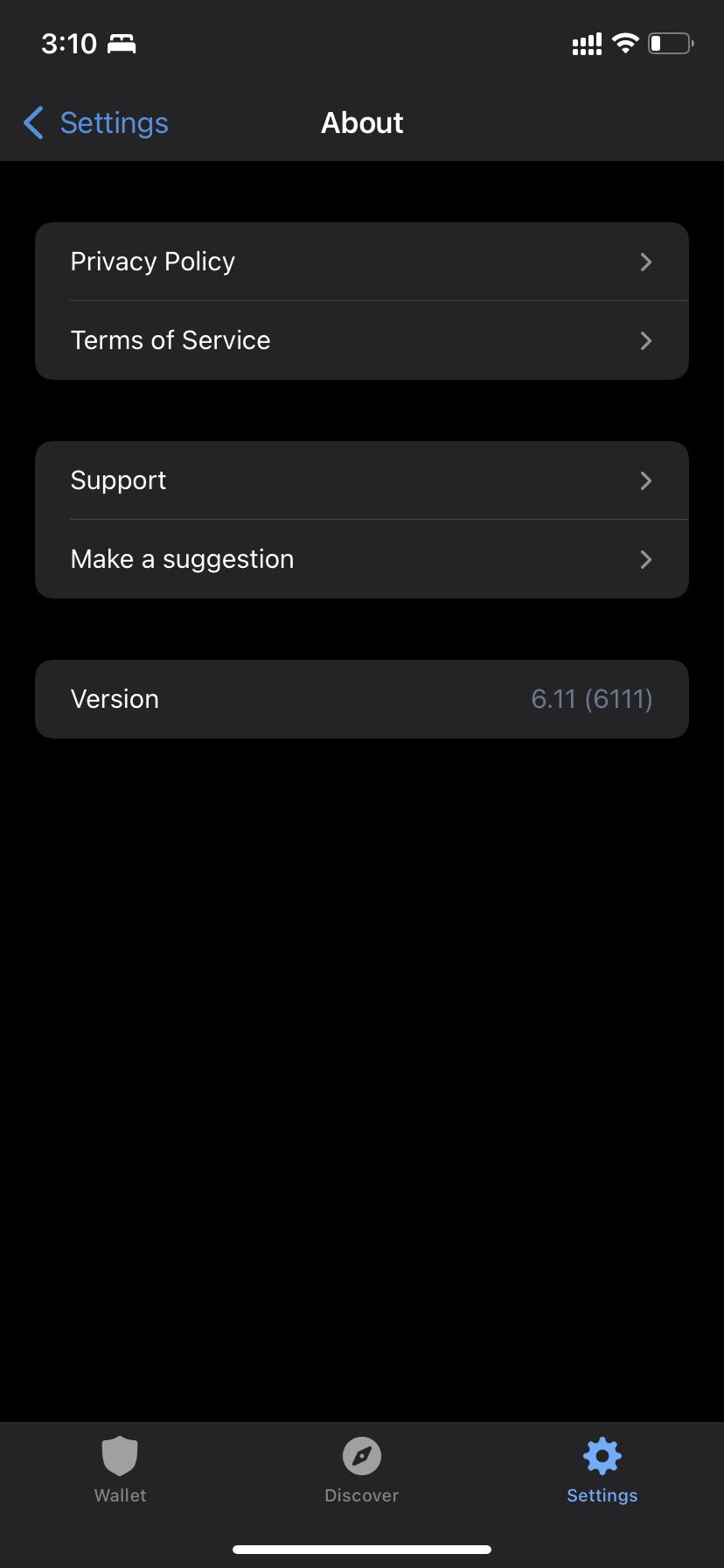A detailed screenshot from an Android phone is depicted. At the top left of the screen, the time reads "3:10," accompanied by an icon right next to it. The top right shows a signal bar at full strength, a full Wi-Fi signal, and a battery icon indicating a quarter charge remaining. Below the status bar, the header section displays "About" in the center, "Settings" with a left-pointing arrow on the left, and “Privacy Policy” followed by a right-pointing arrow, “Terms of Service” with another right-pointing arrow on the right. 

A black space separates these sections from the next: "Area for Support" alongside a right-pointing arrow, and "Make a Suggestion" also with a right-pointing arrow. Another black space further down leads to a rectangular area labeled "Version," containing numbers "6.11 (6111)" in parentheses. 

At the bottom of the screen, three icons are visible: 
1. A wallet icon overlaid with a shield,
2. A discover icon resembling a compass,
3. A settings icon represented by a cog, which is highlighted in light blue.